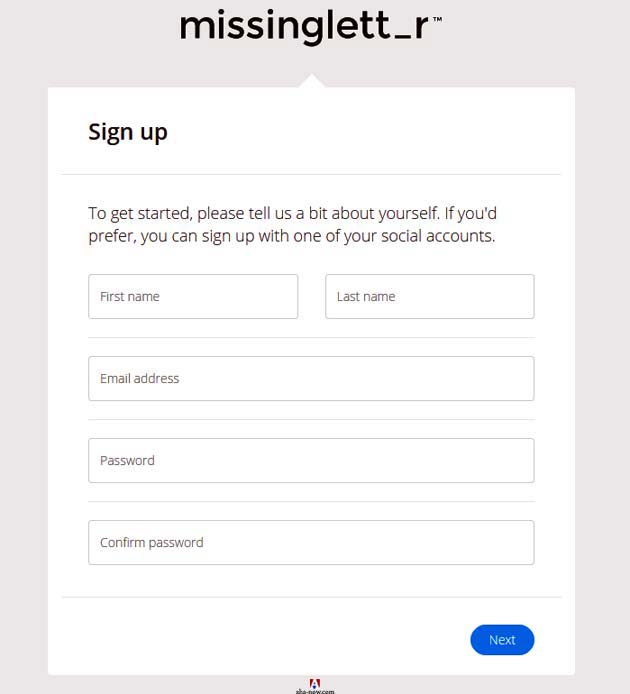This is a detailed caption for an image of a sign-up page:

The image is a screenshot of a sign-up page. Surrounding the central content, there is a light grayish border at the top, left, right, and bottom edges. Centered at the top, the page features the bolded black text "missinglettr_" in lowercase, followed by a small "TM" for the trademark above the "R." Below the "G" in "missinglettr," a small triangular peak spans horizontally, extending about half an inch from the left and right sides, and continues vertically about a quarter inch from the bottom. The background within the border is white.

In the top left corner, bolded black text reads "sign up," underlined by a thin gray line. Below this line, non-bolded black text instructs, "to get started, please tell us a bit about yourself." Another line of text says, "if you'd prefer, you can sign up with one of your social accounts."

Further down, the form contains two white rectangles with black borders: one on the left labeled "first name," and one on the right labeled "last name." Below these fields, there is a thin line, followed by a larger rectangle spanning the page, labeled "email address" in black text. Another line follows, leading to a rectangle on the left side that reads "password" in black, followed by another line and rectangle labeled "confirm password." At the bottom right corner, there's a blue tab with the word "next" in white text.

Finally, at the bottom of the page, a small red square with a white "A" inside is present, accompanied by black text underneath that reads "A something something new dot com."